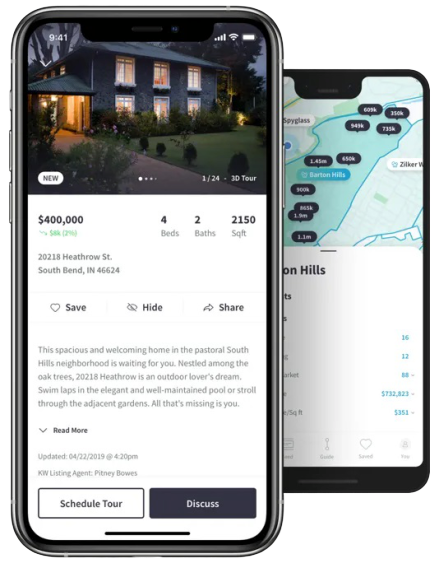In this image, two cell phones display different screens of what appears to be the same real estate app. The larger phone, positioned on top, showcases a listing for a house during what seems to be nighttime or late evening. The majority of the picture is dark, highlighting the house with all its windows warmly glowing. At the top left corner, the time reads 9:41, and the right side displays icons for four bars of mobile data, a strong Wi-Fi signal, and a fully charged battery.

Superimposed on the house picture is an indicator showing 1/24, suggesting there are 24 photos available, along with an option for a 3D tour. The property is listed for $400,000 and features 4 bedrooms, 2 bathrooms, and encompasses 2,150 square feet, located in South Bend, Indiana. Below the image, there's a brief text description with a 'read more' link, and two actionable buttons labeled 'Schedule Tour' and 'Discuss.'

The smaller phone, presumably a different model, displays a map interface with black markers indicating houses for sale. Though much of the textual information is clipped off, the visible location appears to be 'O.N. Hills.'